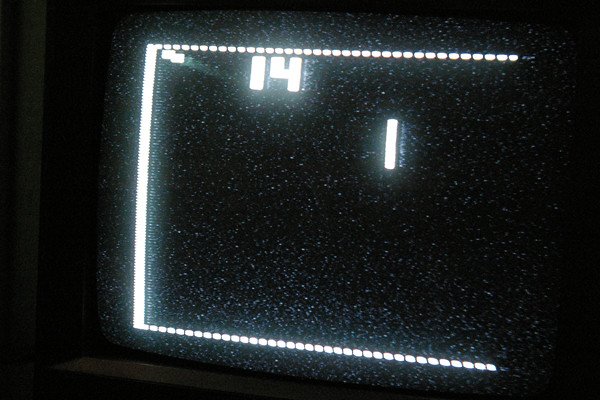The black and white photograph features a nearly black background with a central rectangular screen that appears to display a paused computer or video game. Tiny reflective white specks, resembling stars, are scattered across the screen. Encircling the top, left side, and bottom edges of the screen, there is a series of small, white, rectangular lights. At the top edge, the number "14" is prominently displayed, flanked on the left by two overlapping square lights. Below the "14" on the right side, a vertically oriented, elongated white rectangle is visible. The white specks continue beyond the screen, adding a subtle bluish tinge and blending into the dark background.